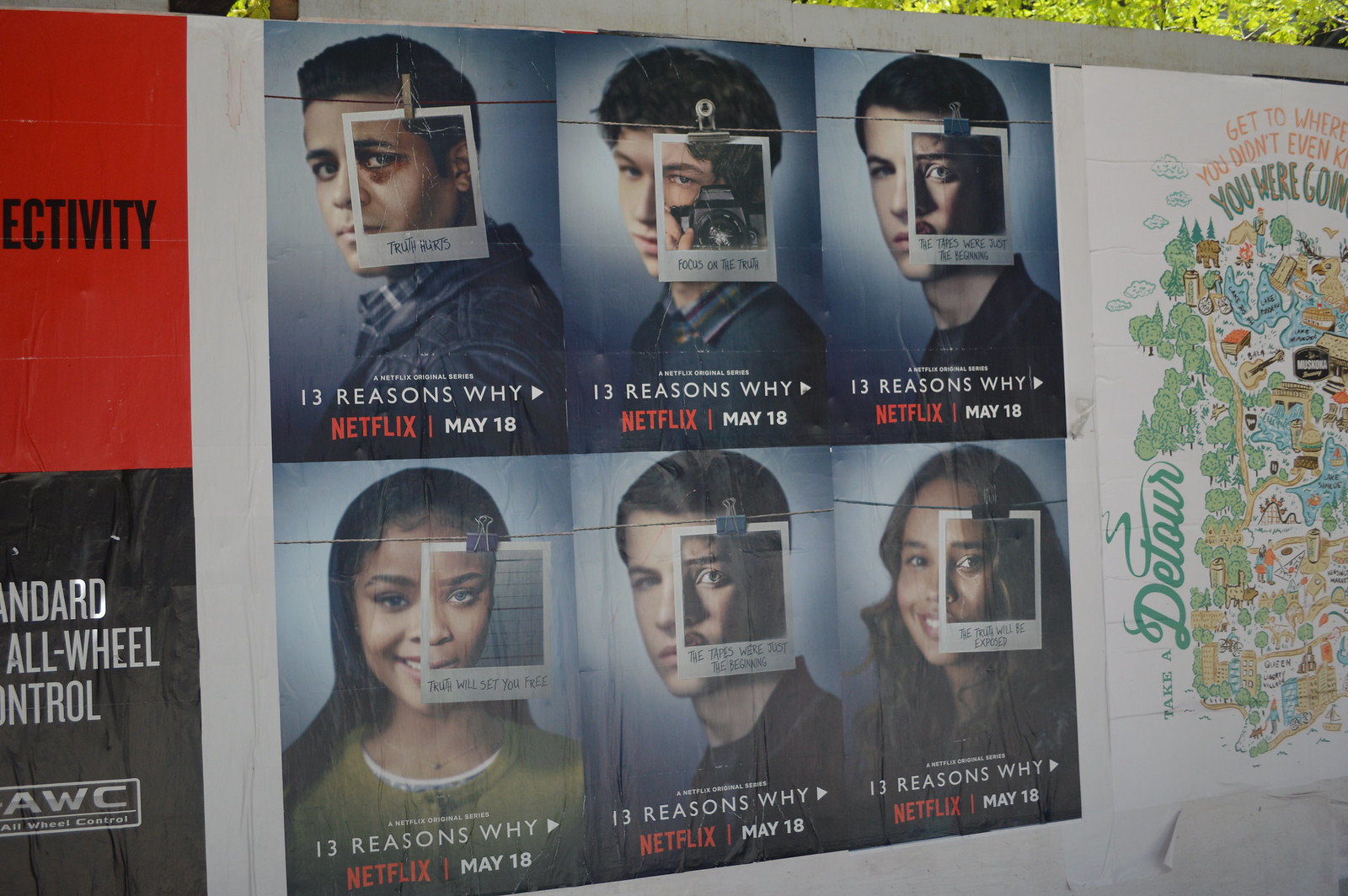This captivating real-life photograph showcases a myriad of posters plastered onto an outdoor wall. The focal point of the image is a series of six prominently displayed posters from the Netflix series "13 Reasons Why," set to premiere on May 18th. Each poster within this main series features a close-up portrait of an individual, framed from the shoulders up, gazing directly into the camera. Intriguingly, the faces of these individuals are partially obscured by Polaroid photos, clipped to red strings with clothespins or paperclips, presenting an altered yet recognizable version of their faces.

The three top posters depict men, all seemingly of Caucasian descent, dressed in casual attire including a jean jacket, a blouse, and a t-shirt. The bottom row portrays a more diverse trio, starting with a black woman in a green blouse, whose Polaroid is uniquely affixed with a paperclip. The next poster features a white male, followed by a darker-skinned female, both continuing the theme of shifted identities through suspended Polaroids. Small, handwritten text appears on these images, though it is too minute to decipher.

Adjacent to this central series, on the right, is a poster filled with illustrations and text. The top part reads, "Get to where you didn't even know you were going," with additional handwritten notes along the side, offering an intriguing but illegible message, potentially "Take a detour." To the left edge of the photo, another poster peeks into view, its top half a striking red and the bottom half black with white text.

The structure that holds these posters is partially visible at the top, revealing a hint of greenery, suggesting an outdoor setting. The bright and natural lighting indicates the photo was taken during the daytime, enhancing the vivid colors and intricate details of the posters.